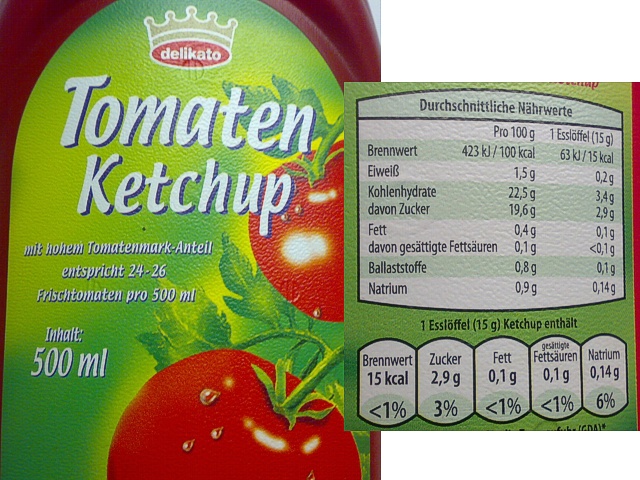This close-up photograph showcases a detailed view of a ketchup bottle label, prominently featuring vibrant colors and intricate design elements. The bottle itself is a striking red with a label that transitions from dark green to a lighter yellow-green towards the center. At the very top of the label, there's a red owl adorned with a slightly grayish crown with small spheres, resembling a delicate crown. Beneath this, the word "Delicato" is displayed in white text, followed by "Tomaten Ketchup" also in large white letters. The image includes two tomatoes on the stem, highlighted with glittery water droplets that reflect light, adding a fresh and appealing look. The left side of the label contains the text in another language, possibly Swedish or Dutch, with additional detailed information provided. The right side of the overall image features a separate green section showing the nutritional information in different languages and numerical values, providing comprehensive details about the product.